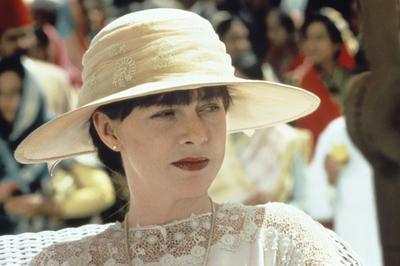The image captures a white woman with short brunette hair, sporting small pearl earrings and dark red lipstick. She is wearing a lace white top and a beige sun hat with a wide brim. She is seated in a white wicker chair, positioned so her shoulders are square to the photo, and she is looking to the right with a slightly annoyed expression. The setting is ambiguous, as it's unclear whether it's indoor or outdoor, daytime or nighttime. Behind her is a blurred background depicting what appears to be a large crowd, possibly a mural, with indistinct figures displaying various colors such as red, gold, brown, off-white, teal or blue, and tan. The woman is almost entirely in the frame, with the background elements remaining indistinct and secondary to her presence.